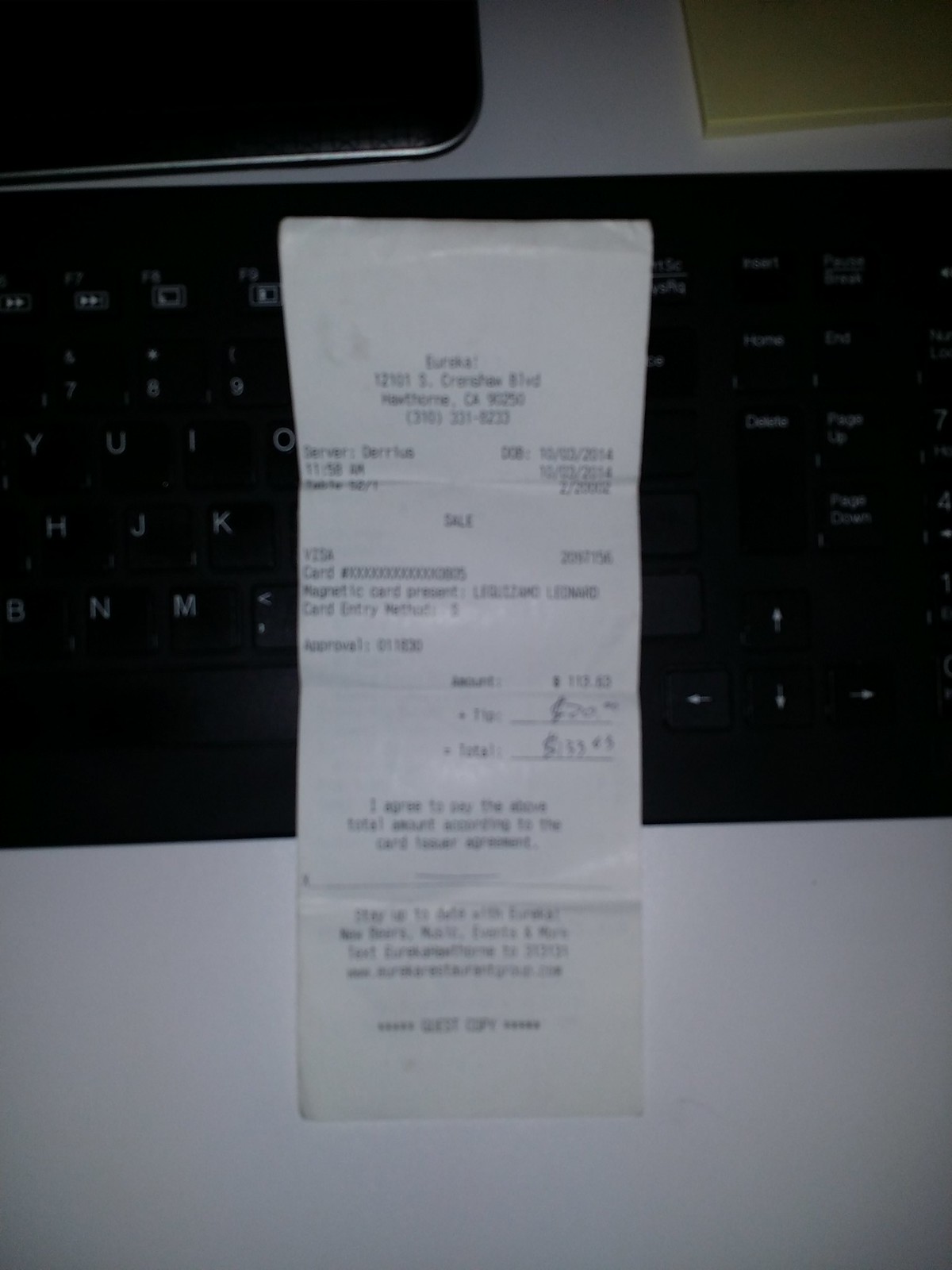In this image, a slightly out-of-focus white paper receipt is laid on top of a silver-paneled laptop. The receipt displays a typical format, featuring sections for the total amount, tip, and a final total. However, the text and numbers on the receipt are too small and blurred to be readable. The focal point shifts to the laptop's keyboard, where specific black keys with white lettering are clearly visible, including the characters Y, U, I, O, H, J, K, N, and M, along with directional arrow keys.